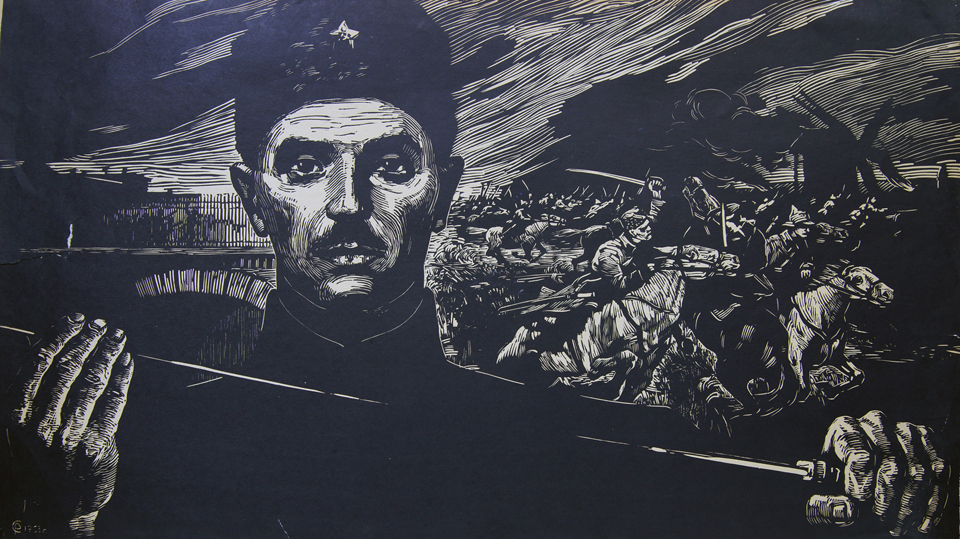This is a detailed black and white pen and ink illustration, possibly a lithograph, depicting a chaotic battle scene. In the foreground stands a stern-faced man, presumably a Cossack, identifiable by the distinctive star on his thick, furry hat. He sports a mustache and is dressed in a dark military uniform. The man holds a sword in both hands, the blade angled towards the upper left part of the image. Below his right ear, there's a bridge with a fence. Swirling, dark clouds stretch across the sky, creating a stark, tumultuous backdrop. Behind the man, to his left and right, soldiers on horseback with swords raised are galloping off, vividly capturing the intensity and motion of an ongoing battle.